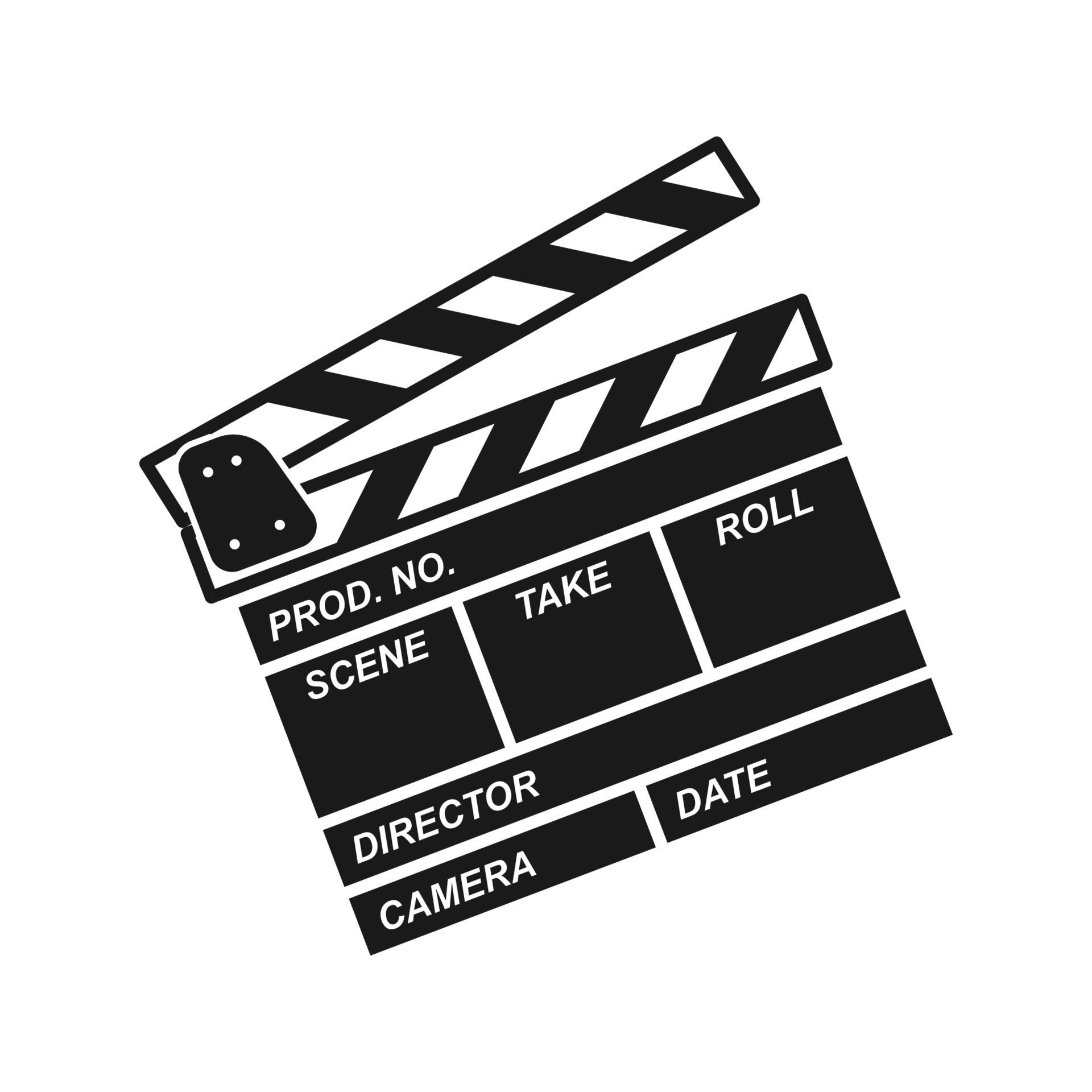The image depicts a black-and-white cartoon-style drawing of a clapperboard, set against a plain white background. The clapperboard, commonly used in film production to mark scenes and takes, features sections labeled "Prod No", "Scene", "Take", "Roll", "Director", "Camera", and "Date." Each section is designed to be written on using chalk. The image highlights the traditional components of a clapperboard, including the hinged top that snaps open and shut, used to signal the start of recordings with a distinctive clapping sound.